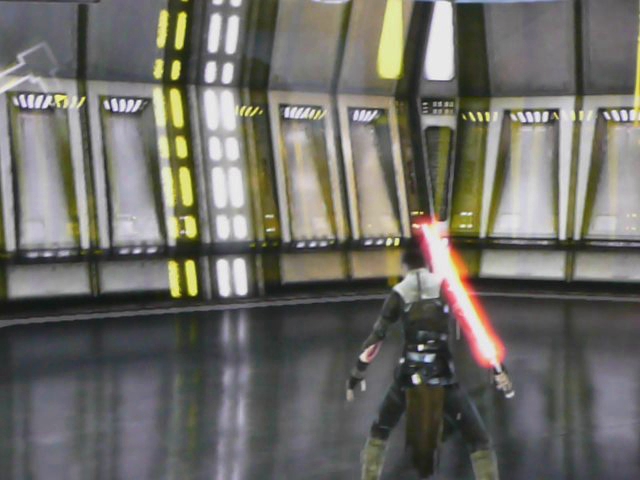A person stands against a highly reflective black floor, holding a red lightsaber behind their back in their right hand. The individual is dressed in black pants and brown shoes, with a cloth draped to the bottom. Their left arm has a noticeable cut on the forearm. The person has short hair and a white shirt. The surrounding area features white, curved walls that rise upward and are divided into sections by metal braiding. On the middle left side of the scene, yellow ovals rise upward alongside white ones, separated by more sectioned spaces. Above, a yellow light and a white light are visible, adding further illumination to the space.